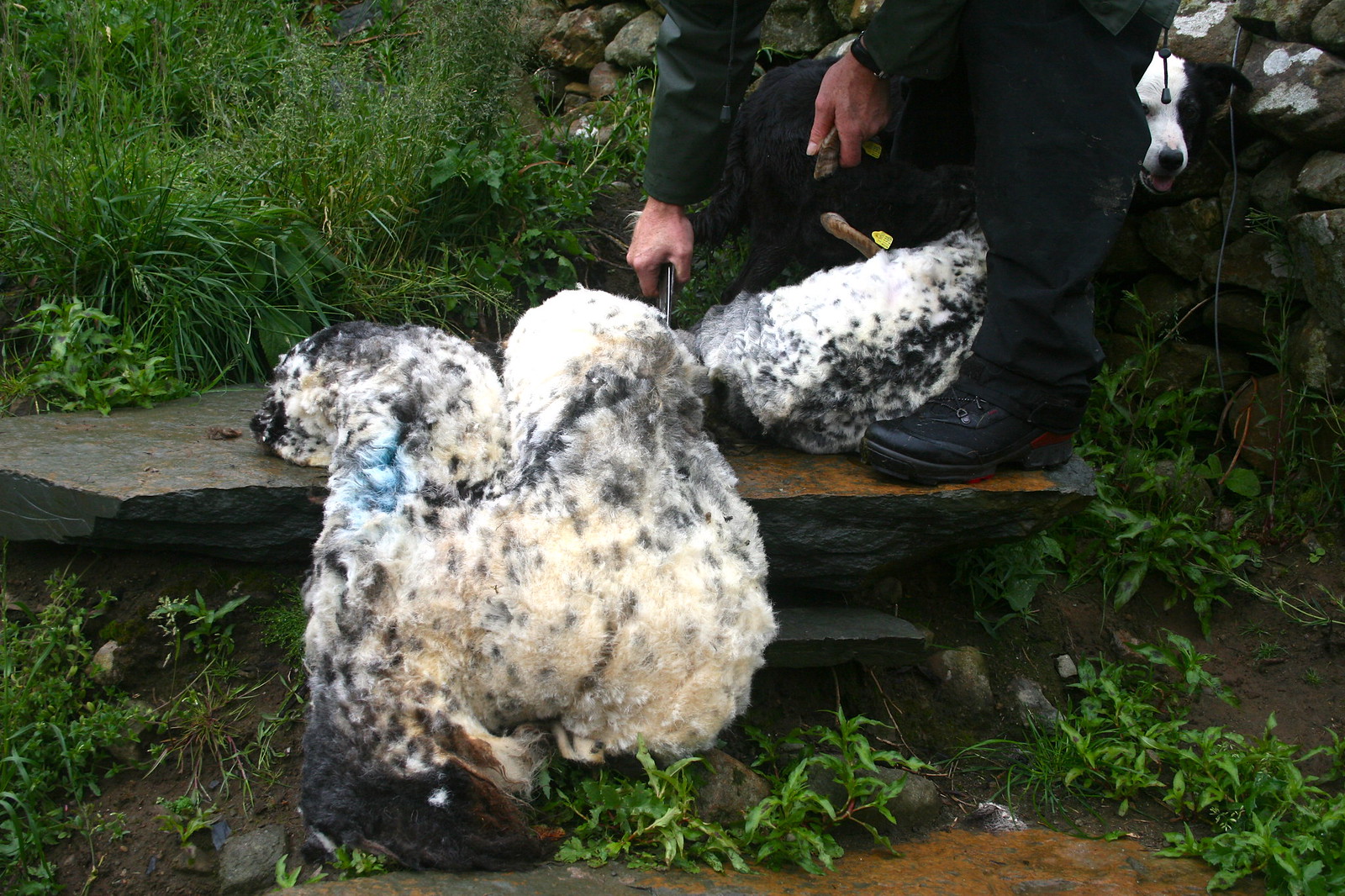In this color landscape photograph, we see a detailed outdoor scene featuring a moment of animal shearing. At the center of the image, a largely white sheep with black and gray speckling lies on a dark gray, wet-textured stone ledge, which has some orange hues near the top. The sheep's head rests on the ground, and its body stretches across the rocky step. Above the sheep, a person, whose upper body and face are cut off from the frame, is seen standing with black sneaker-style shoes and black pants. In their right hand, they hold a shearing implement.

The environment appears recently rained upon, giving everything a slick, wet sheen. A thick mat of sheared wool sits at the person’s feet, suggesting that the shearing is underway or recently completed. In the scene's upper portion, there is deep, lush green grass interspersed with patches of sparse areas where the grass is less dense. In the top right corner, a partial view of a black and white dog peeks from behind the person’s legs, adding to the pastoral ambiance. Another dog with predominantly white fur and some black and gray speckling is also present, contributing to the lively snapshot of rural life.